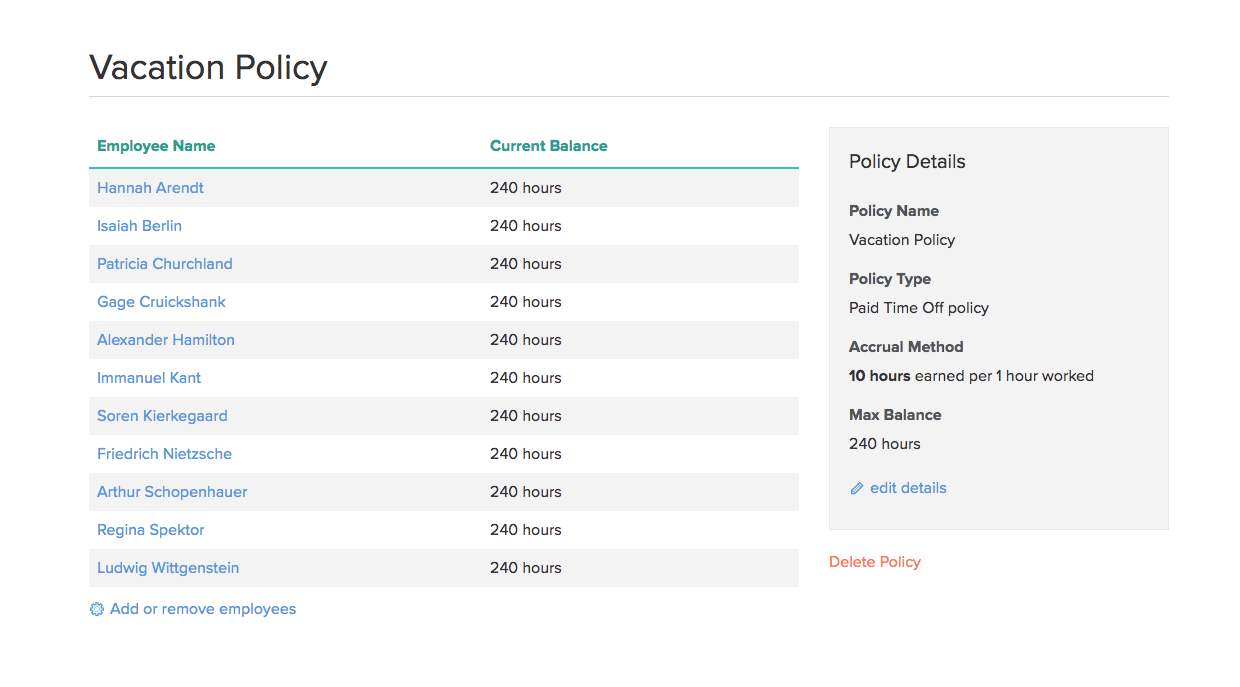The image is a cropped screenshot showcasing the "Vacation Policy" tab on an HR software interface. At the top left, "Vacation Policy" is prominently displayed in very large black font against a white background. Directly under this title, a thin gray line extends horizontally across the entire page.

Beneath this line is a boxed section with horizontal rows alternating in gray and white. Each row lists an employee's name to the left, followed by a number indicating their vacation hours to the right. The first row highlights Hannah Arendt in a gray box with a current balance of 240 hours of vacation time. This pattern continues alternately, with the next name in a white box and so forth, each indicating a balance of 240 hours. 

To the right of the employee section is a large gray box labeled "Policy Details" at the top. This box contains several specifications:
- "Policy Name" with the value "Vacation Policy"
- "Policy Type" listed as "Paid Time Off Policy"
- "Accrual Method," which specifies "10 hours earned per 1 hour worked" (with "10 hours" and "1 hour" in bold)
- "Max Balance" set to "240 hours"

At the bottom left of this box, there's a blue "Edit Details" section, and "Delete Policy" is written in small red letters just below to the left.